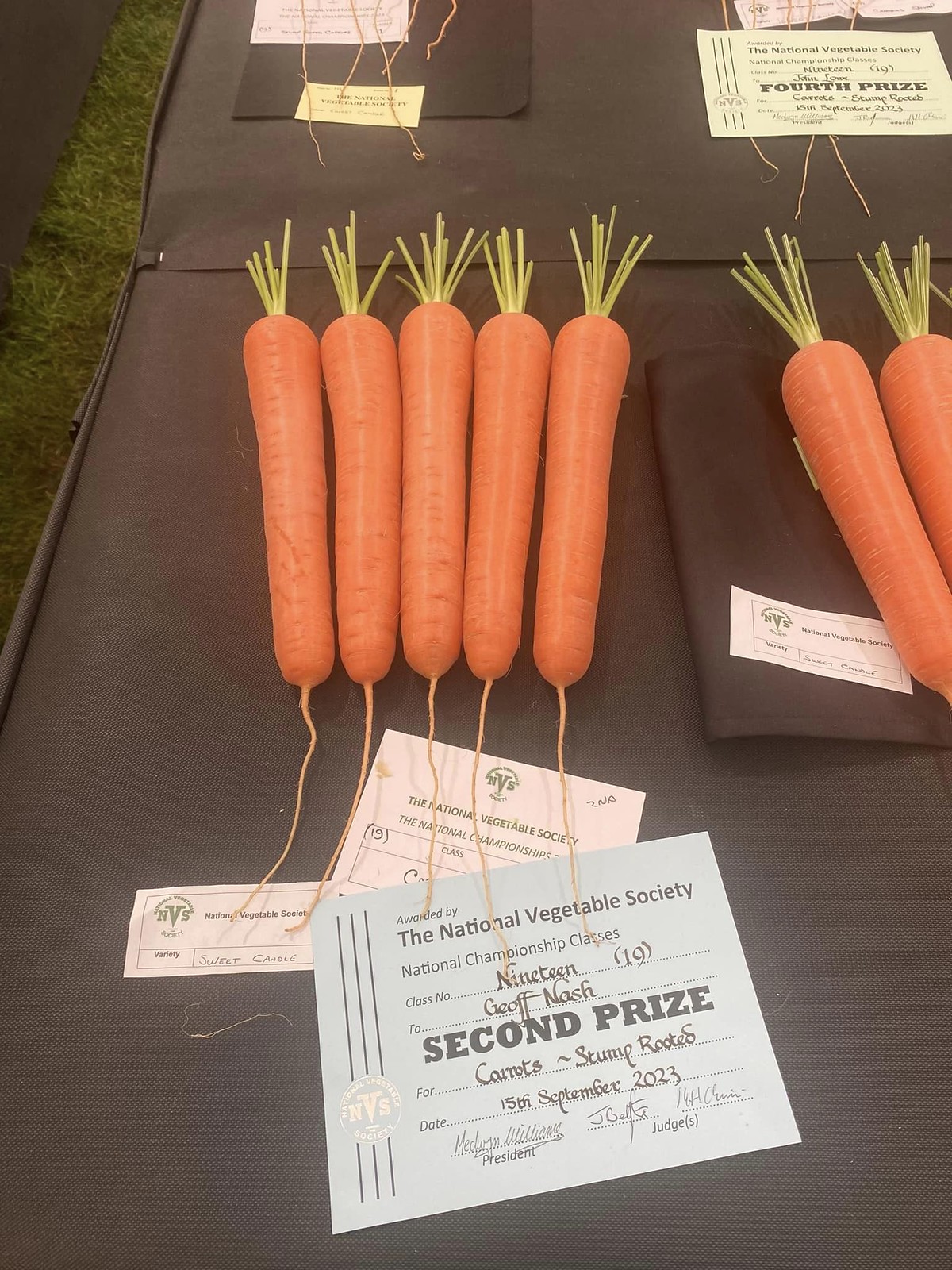The photograph captures an image taken at a National Vegetable Society competition, likely the National Championships, on a grassy field. Central to the image are five almost identical, perfectly shaped carrots laid out on a brown tarp or mat. These carrots are notable for their vibrant orange color, uniform size and shape, and straight green tops with tiny, thin roots. Beneath the main set of carrots, there's a blue placard that reads: "Awarded by the National Vegetable Society, National Championship Classes. Class number 19 to Jeff Nash, Second Prize for Carrots (Stump Rooted). Date: 15th September 2023." This placard also features signatures from the president and judges. To the right of this main display, a second pair of carrots is partially visible, and above this, a yellow placard denotes a fourth prize in a different class. Additional illegible placards are scattered around the tarp. The scene suggests a well-organized, prestigious event with a detailed judging and awarding process.